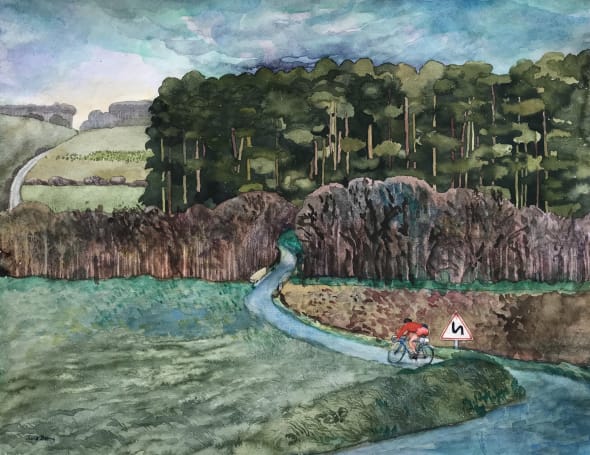This watercolor painting captures a picturesque outdoor scene featuring a winding pathway that meanders through a richly detailed landscape. The pathway, which resembles a bike trail, leads from the foreground into the distant woods. A sign with a curved arrow indicates a bend in the road, emphasizing the pathway's serpentine nature. A lone cyclist, dressed in red, is midway along the path, surrounded by an array of natural elements. 

On the left side of the image, the landscape features green fields extending into the distance, punctuated by some bare trees. To the cyclist's right, the terrain shifts to a brownish field leading up to a dense forest. The forest is composed of both smaller, brown trees in the foreground and towering green trees behind them, creating a layered effect that enhances the depth and richness of the scene. 

Above, a light blue sky with scattered, bumpy clouds—shaded in hues of blue and green—caps the composition, occupying the uppermost part of the painting. The sun's influence is subtly indicated by a lighter patch in the sky on the left. 

Overall, the painting is dominated by a harmonious blend of greens, tans, and blues, with the watercolor technique giving a fluid, blended quality to the colors, further enriching the natural ambiance of the scene. Whether it depicts a forest or a park, the detailed depiction of the flora, the meandering path, and the solitary cyclist invite viewers into a tranquil, verdant world.